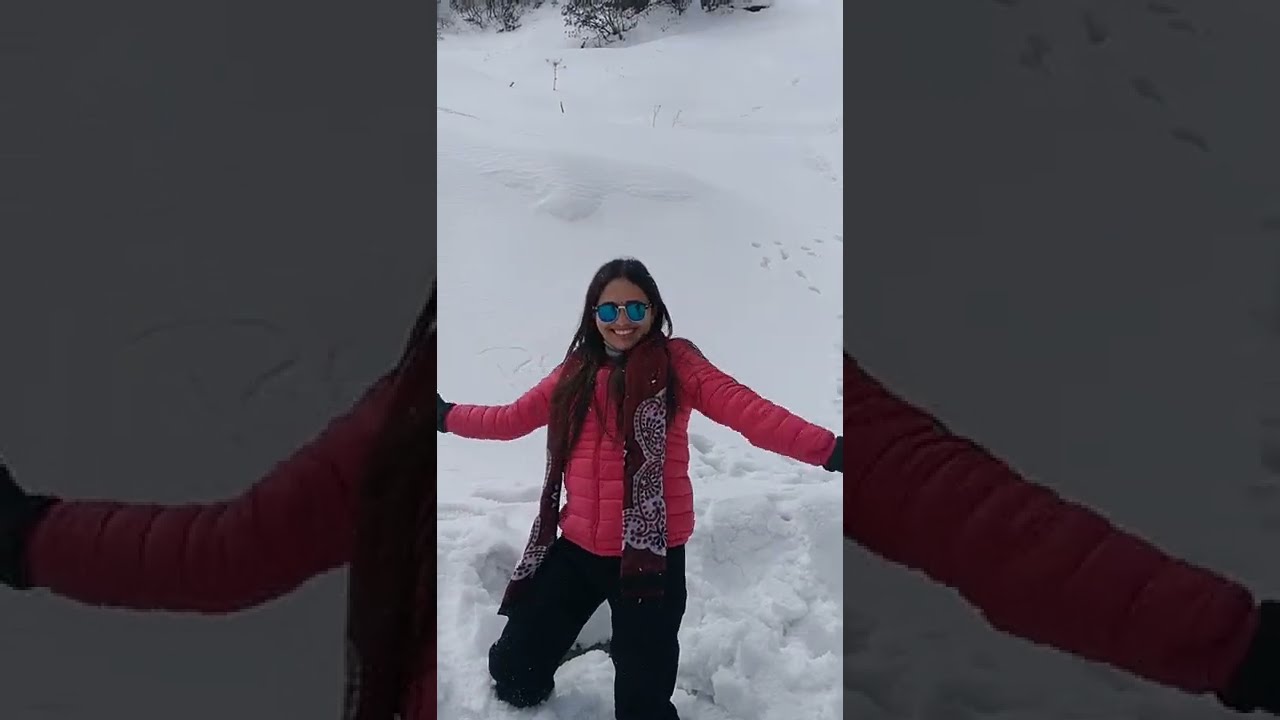The central image captures a young woman with dark brown skin and long dark hair, which almost reaches her waist, standing in a snowy landscape. She wears blue-tinted sunglasses and smiles widely, revealing her teeth. She is dressed in a puffy red winter coat that extends to her wrists, a maroon scarf with white embroidery around her neck, black gloves, and black pants. She stands on a pile of snow, with snow rising uphill into some bushes at the top of the image. Her arms are outstretched to either side, slightly overlapping the left and right columns, which are zoomed-in and faded sections of her left and right arm, respectively. The snow around her is disturbed, with noticeable footprints leading towards her.